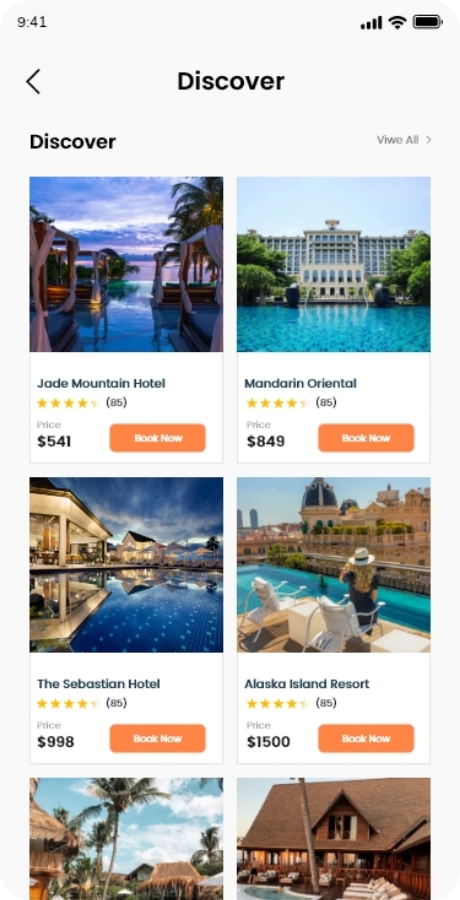Screenshot of a smartphone displaying hotel booking options. The top left corner shows the time, while the right corner features the Wi-Fi symbol and battery percentage. The screen displays the title "Discover," alongside various hotel listings with accompanying images.

- **Top Listing**: 
  - *Jade Mountain Hotel*: 
    - Image: Showcases a luxurious water resort.
    - Rating: 4.5 stars based on 85 reviews.
    - Price: $541 per night.
    - Action: Orange "Book Now" button.

- **Second Listing**: 
  - *Mandarin Oriental*:
    - Rating: 4.5 stars from 85 reviews.
    - Price: $849 per night.

- **Third Listing**: 
  - *The Sebastian Hotel*:
    - Rating: 4.5 stars based on 85 reviews.
    - Price: $998 per night.

- **Fourth Listing**: 
  - *Alaska Island Resort*:
    - Rating: 4.5 stars based on 85 reviews.
    - Price: $1500 per night.

Additional images at the bottom depict potential stay options:
- One image shows an area lush with palm trees and open outdoor space.
- Another image displays a cabin-like structure resembling a traditional home with a pool area.

Overall, the screenshot appears to be from an app used for booking stays at hotels or other rental properties.